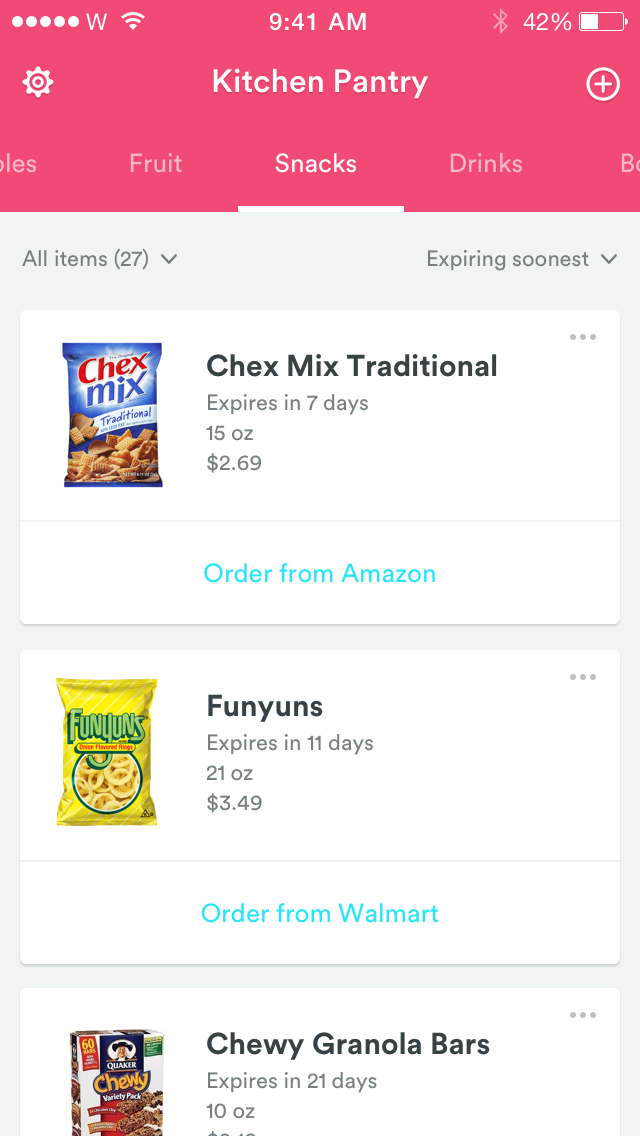The screenshot of a cell phone, taken at 9:41 AM, shows the device connected to Wi-Fi with 42% battery remaining and Bluetooth enabled. The screen displays a digital kitchen pantry application. At the top of the app interface, there is a settings sprocket and a plus sign for adding items. Listed categories include Vegetables, Fruits, and Drinks, with "Snacks" currently highlighted among them. The app also offers sorting options, showing all 27 snack items with the ability to sort by "expiring soonest."

The first item displayed is Chex Mix Traditional, which comes in a 15-ounce package priced at $2.69 and expires in seven days. There is an option to order it from Amazon, accompanied by a picture of Chex Mix. The next item is a bag of Funyuns, weighing 21 ounces and costing $3.49, which expires in 11 days and can be ordered from Walmart. Finally, the last listed snack is a pack of Quaker Chewy Granola Bars, weighing 10 ounces, and expiring in 21 days, though the price is partially cut off in the screenshot.